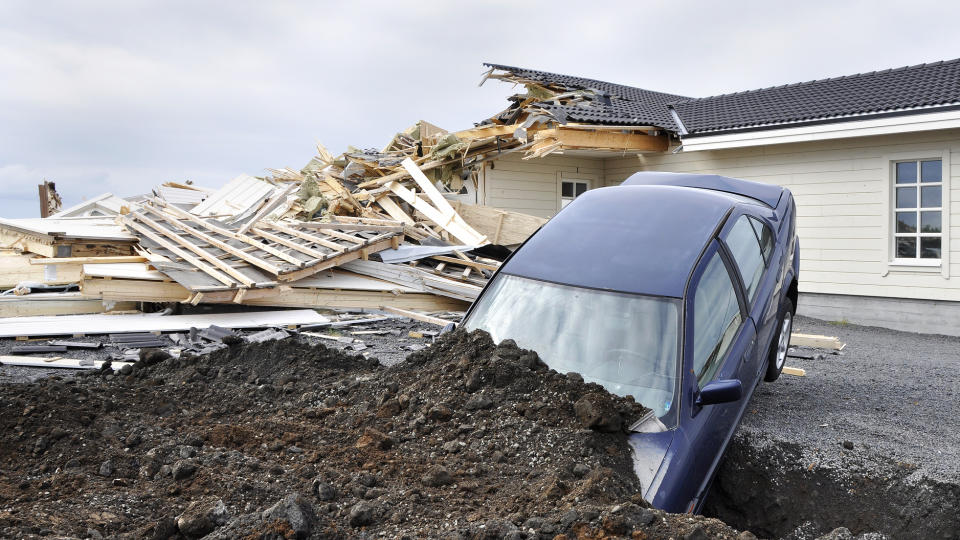This image captures the devastation left in the wake of a catastrophic event. Dominating the background is an L-shaped, pale yellow house. While the right side of the house remains intact, the left side has been obliterated, reduced to a chaotic pile of rubble with only partial sections of the roof still visible among the disarray of lumber and loose boards. 

In the foreground, a car precariously nose-dives into a crevice, its hood buried and windshield partially obscured by debris. The vehicle is angled sharply downward toward the camera, with its rear wheels suspended above the rough, uncovered dirt. The crevice continues off to the right, adding to the scene's sense of upheaval. 

Above, the sky contrasts sharply with the destruction below, painted in a serene blue adorned with fluffy white clouds, creating a stark juxtaposition between the tranquility of the heavens and the chaos on the ground.